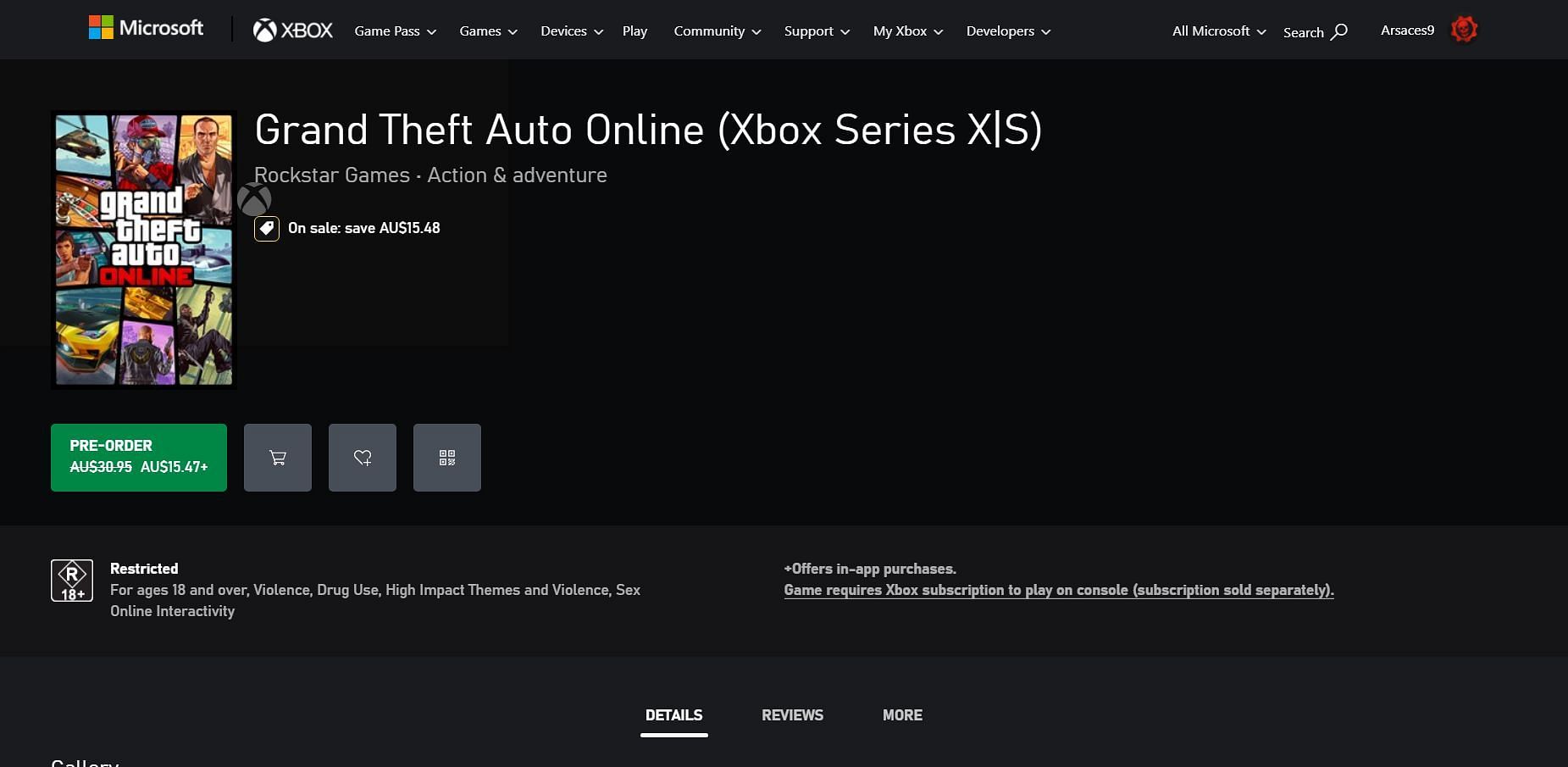This image captures a screenshot of the Microsoft Xbox Game Store, showcasing the pre-order page for "Grand Theft Auto Online." The interface appears to be consistent whether accessed from an Xbox console on a TV or from a computer, featuring a predominantly black background. Central to the screen is the cover art of "Grand Theft Auto Online," mimicking what one might see on a physical game case. To the right of the image, text displays critical information: "Grand Theft Auto Online - Xbox Series X|S - Rockstar Games - Action & Adventure." Above, a header bar is replete with various drop-down menus for navigating the Game Store. At the bottom of the screen, there is an indication that more game details can be scrolled into view. The page includes essential interactive buttons such as "Pre-order," highlighting the primary call to action.